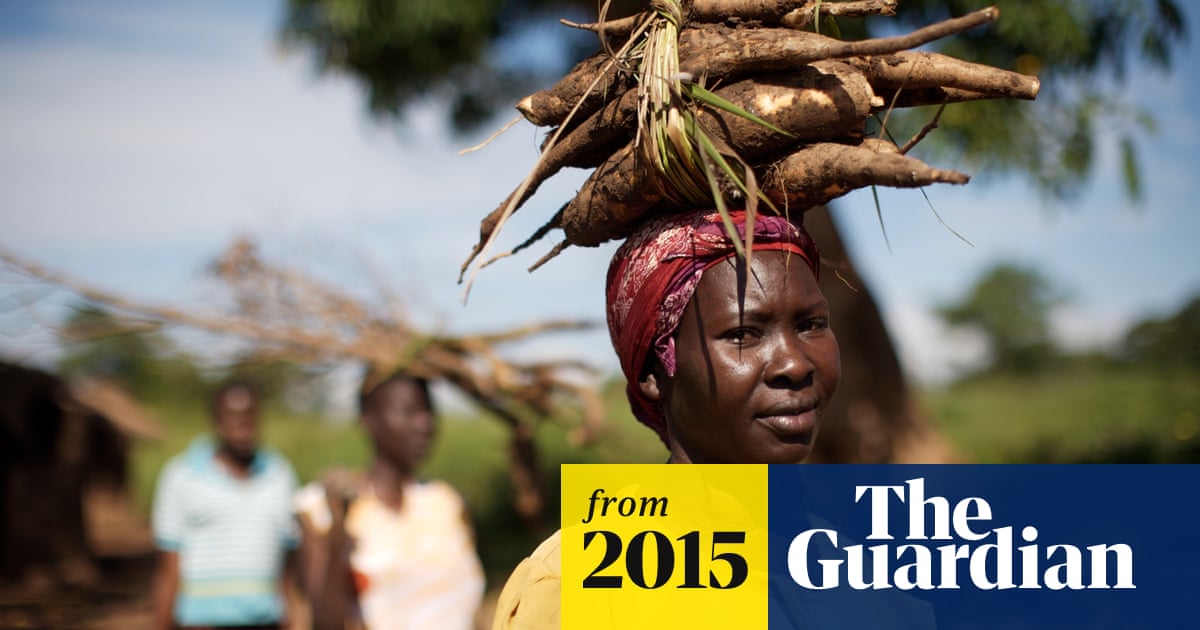The photograph, taken outdoors and set against a blurred backdrop of a blue sky and green canopy leaves, features a young African woman in her early 20s carrying a bundle of large, brown, oval-shaped root vegetables, possibly yams or a similar tuber, secured with a bundle of grass atop her head. She is facing right, bathed in sunlight that glistens on her dark skin, with a relaxed smile on her face. Her head is wrapped in a red, purple, and white printed scarf, with two wisps of hair peeking out over her forehead. Positioned prominently in the foreground, she is the focal point of the photograph. In the background, albeit blurred, there are two other individuals of African descent: a woman wearing a white sleeveless top also balancing items on her head and a man in a short-sleeved blue shirt. Both background figures are out of focus, adding depth to the scene. Positioned in the lower right corner of the image is a horizontal graphic bar, with the left side in bright yellow bearing the text "from 2015" in dark blue serif print, and the right side in dark blue with bold white serif text reading "The Guardian."